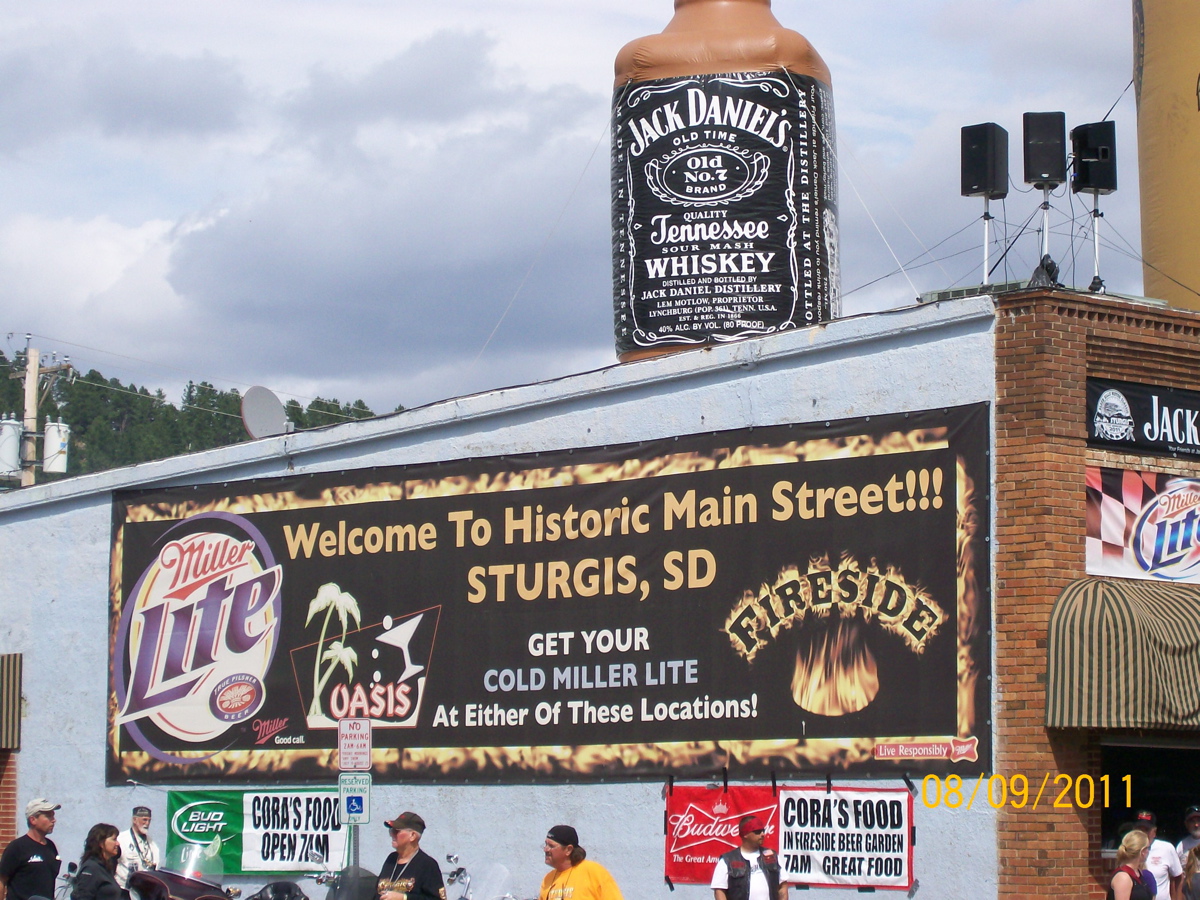This detailed photograph, dated August 9, 2011, captures the bustling exterior of a building situated on the historic Main Street of Sturgis, South Dakota. The building, which appears to be either a bar or a liquor store, showcases a striking contrast between its reddish-brown brick front and its light blue painted side wall. Dominating the side wall is a large rectangular banner bordered by fiery flames, with "Welcome to Historic Main Street, Sturgis, SD" prominently displayed. Beneath this greeting, it advertises cold Miller Lite available at "Oasis" and "Fireside," with the Miller Lite logo positioned on the left side of the banner. Adjacent to this, the word "Oasis" is illustrated alongside palm trees and a martini glass, while "Fireside" is introduced as a beer garden that serves great food from 7 a.m., accompanied by a Budweiser logo.

Further accentuating the celebratory ambiance, a giant inflatable Jack Daniels Tennessee Whiskey bottle with its iconic black label and white font sits on the roof of the building, near some mounted speaker stands. At street level, the scene depicts a lively parking lot filled with people, many of whom are gathered near their motorcycles, enhancing the image's quintessential biker culture vibe.